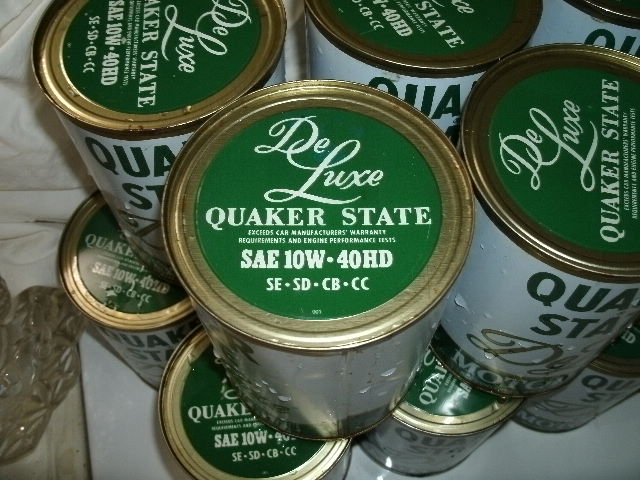This photo features a stack of vintage oil cans, primarily colored white and green. The cans are adorned with green lids, each encircled by a yellow outer rim. The top of each can is emblazoned with the text, "Deluxe Quaker State," followed by a detailed description: "Exceeds car manufacturer's warranty requirements and engine performance tests. SAE 10W-40HD-SE-SD-CB-CC." The cans are meticulously arranged one on top of the other, creating a symmetrical tower-like structure. Notably, several cans exhibit water droplets, suggesting recent exposure to moisture or condensation. The entire arrangement rests on a polished marble floor, adding a touch of elegance to the display.